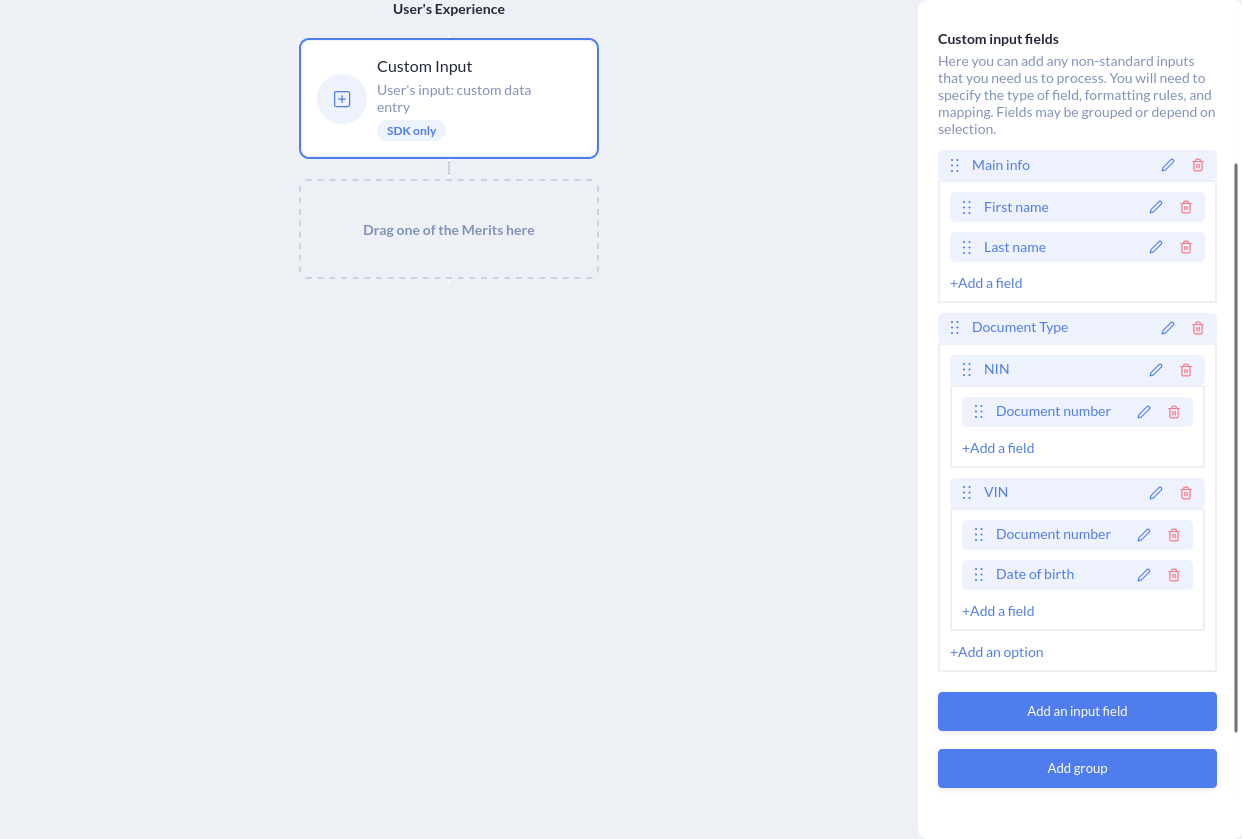This image is a screenshot from an unidentified source. The left side of the screenshot features a solid gray background. At the top of this section, the text "User's Experience" is prominently displayed. Below that, there's a white rectangle outlined in blue, containing various labels: "Custom Input," "User's Input," "Custom Data Entry," and "SDK Only." Extending downward from the bottom of this blue-outlined rectangle is a thin, vertical line that connects to another rectangle made up of dotted lines. Inside this dotted rectangle is the instruction: "Drag one of the merits here."

To the right of the gray area, there's a vertical section labeled "Custom Input Fields." This area includes explanatory text: "Here you can add any non-standard inputs that you need us to process. You will need to specify the type of field, formatting rules, and mapping. Fields may be grouped or depend on selection." Below this text, the section is divided into several input fields labeled "Main Info," "First Name," "Last Name," along with options to "Add a Field." Additional categorizations for input fields include "Document Type," "NIN," "Document Number," "VIN," "Document Number," "Date of Birth," with corresponding buttons to "Add a Field" and "Add an Option." 

At the bottom of this section, there are two blue rectangles: one labeled "Add an Input Field" and the other "Add Group."

The screenshot lacks any photographic elements, such as people, animals, plants, flowers, or trees. It's purely a graphical user interface design, focusing on data entry and customization options for user inputs.